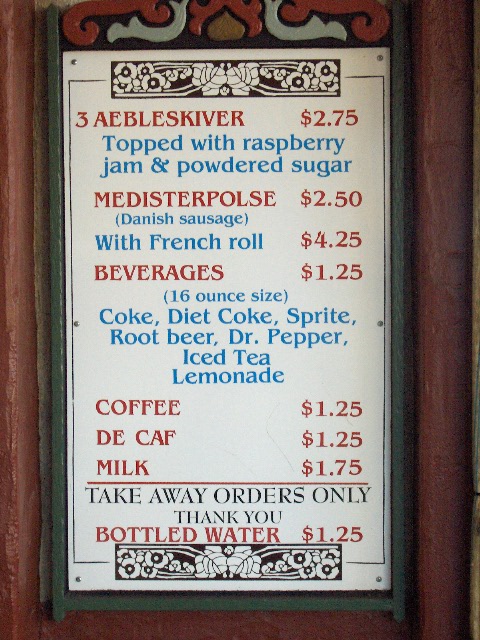A rustic and intricately crafted wooden frame, characterized by its rich brownish-red hue, encases a charming menu. The frame features delicate colored glass accents in shades of reddish, gray, and brown, adding a touch of elegance as it suspends the menu in mid-air. The menu itself is printed on white paper and adorned with a whimsical black drawing at the top, depicting white flowers with black centers, arranged to form a butterfly-like shape in the middle.

The menu items are listed in a mix of red and blue writing. At the top, written in red, is "Three Æbleskiver" priced at $2.75, with a description in blue stating they are "topped with raspberry jam and powdered sugar." 

Next, in red, "Matister Pulse" is listed for $2.50, followed by a blue description of "Danish Sausage with French Roll" for $4.25 in red text.

Under the beverages section, in red, the menu lists drinks for $1.25, with blue text specifying a "16 oz size" for Coke, Diet Coke, Sprite, Root Beer, Dr. Pepper, Iced Tea, and Lemonade. Coffee and decaf are both listed at $1.25 in red, accompanied by milk at $1.75. 

A bold red line demarcates a section with the following black text: "Takeaway orders only. Thank you." Finally, the menu mentions bottled water, priced at $1.25 in red.